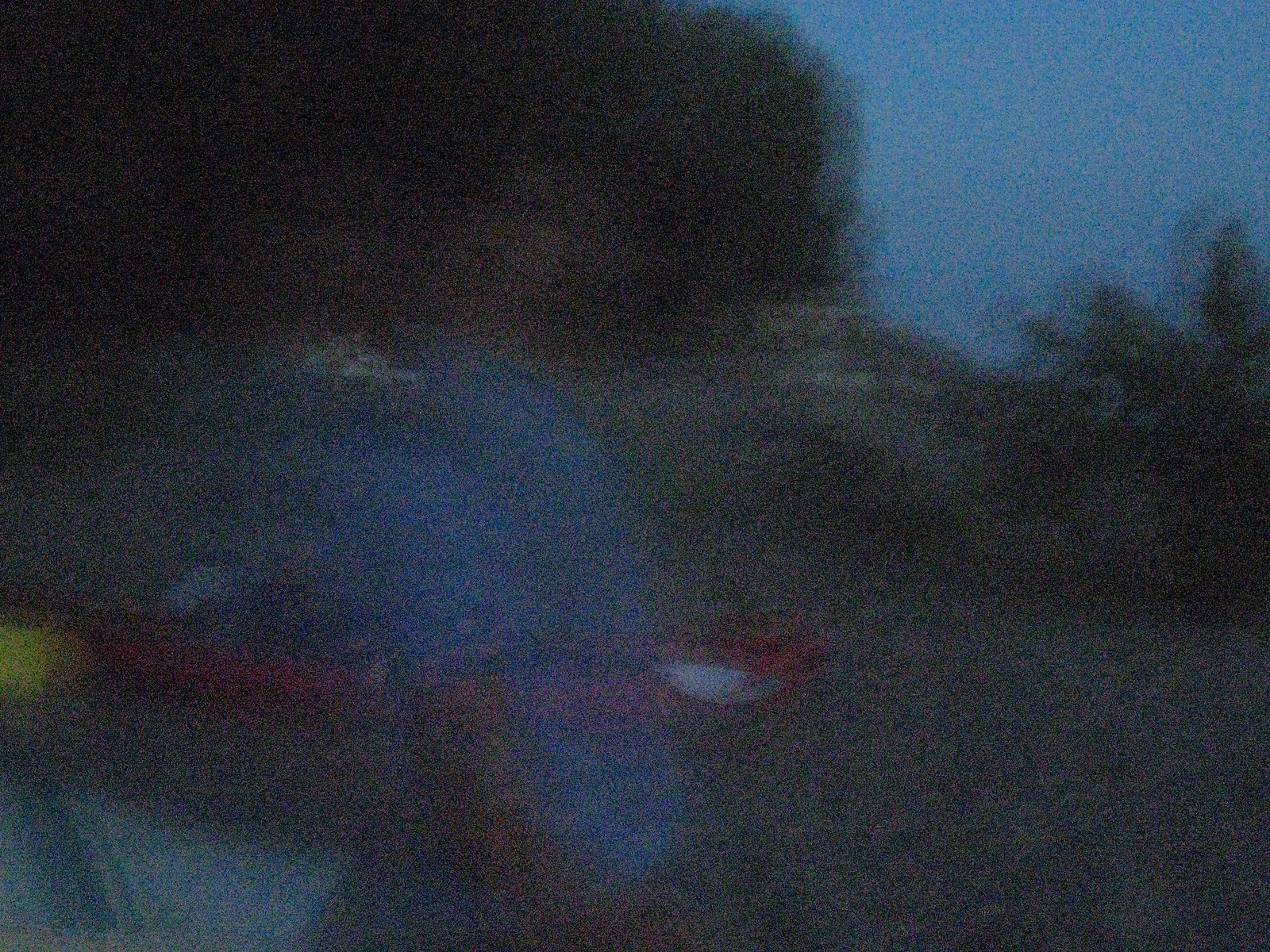This extremely blurry photograph appears to capture a scene in someone's yard at night. On the right side of the image, dark-colored trees and bushes blend into the shadowy surroundings, while the inky night sky adds to the obscurity. Moving to the left side, the poorly-lit scene reveals what might be a children's yard toy, possibly a teeter-totter, characterized by its dark red color and what appears to be a bucket seat. The foreground looks gravelly, and there seems to be a bluish tent-like object with a red base, suggesting an open flap typical of tent doors. The low quality and dim lighting of the image make it challenging to distinguish these elements clearly, lending an almost ghostly effect to the hues of green, blue, and red that punctuate the otherwise dark and amorphous scene.